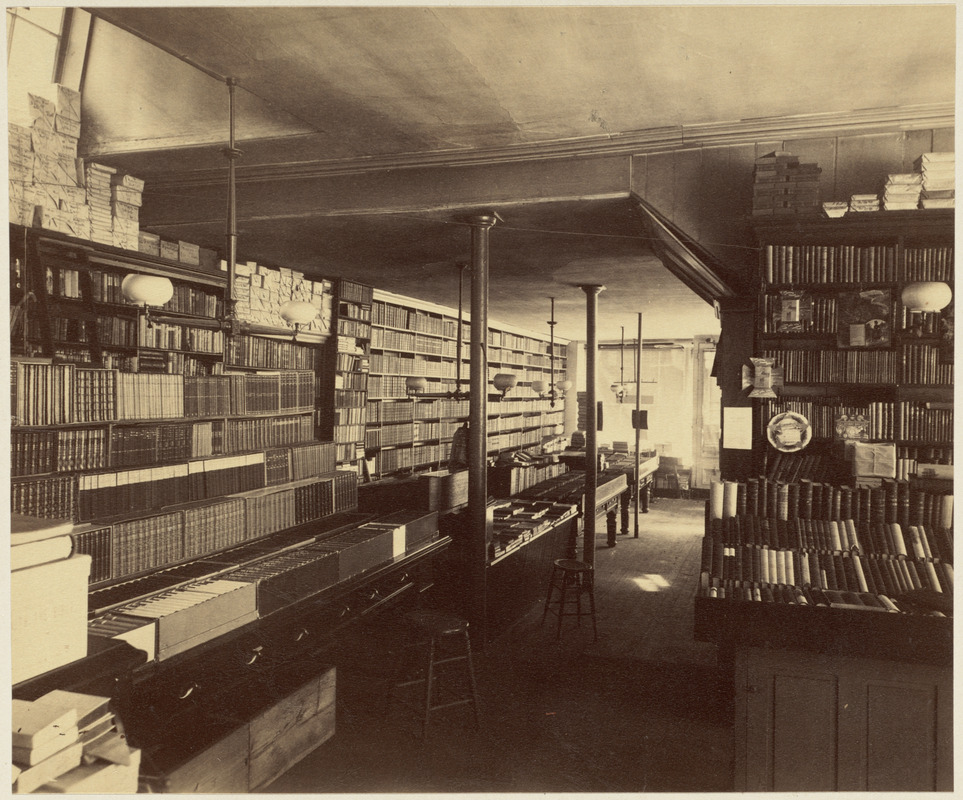This vintage sepia-toned photograph captures a meticulously organized small-town library or bookshop, likely from the early to mid-20th century. The image features tall wooden shelves brimming with neatly stacked hardcover books, arranged alphabetically and free from any disorganization. The library's interior showcases wooden cabinets and two prominent wooden columns supporting the ceiling. In the center, there are tables with large encyclopedias, their thick stems adorned with silver trimmings. The room also has a counter, possibly with a glass partition, contributing to the quaint, timeless atmosphere. The absence of people and the yellowish tint of the photograph enhance its historic ambiance, making it a perfect snapshot of a bygone era's literary haven.